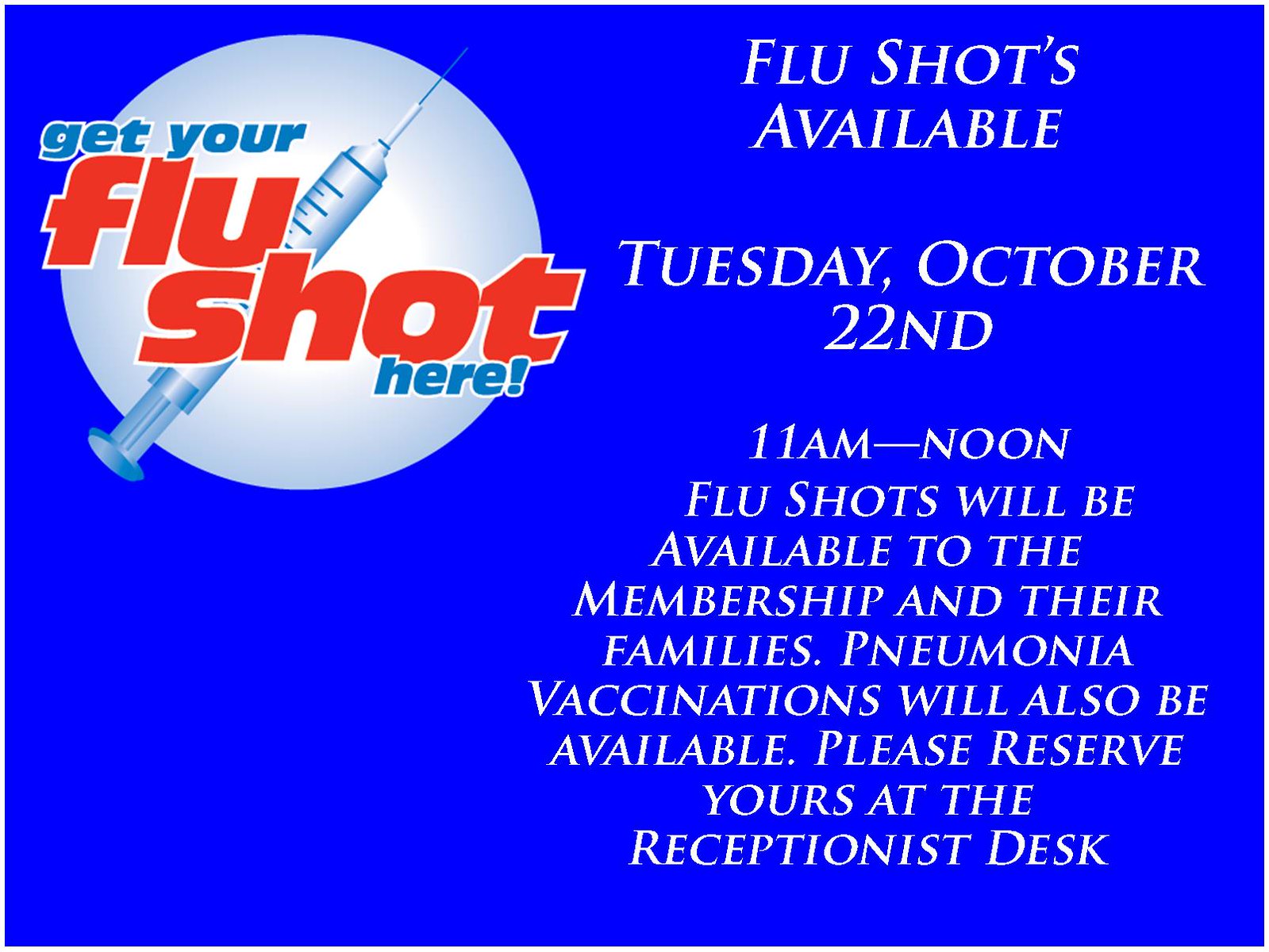This image is a detailed advertisement for flu shots designed with a royal blue background. In the top left corner, there is a white circle containing a graphic of a syringe angled upwards at 45 degrees, with red text that reads "Get Your Flu Shot Here." Below this logo, the main information is presented in white text, which states: "Flu shots available Tuesday, October 22, 11 a.m. to noon. Flu shots will be available to the membership and their families. Pneumonia vaccinations will also be available. Please reserve yours at the reception desk." The font used is serious and official, resembling Times New Roman, and is entirely in capital letters, providing a clear and formal announcement. This structured layout of text and imagery ensures the viewer's attention is drawn to the important details of the vaccination offering.